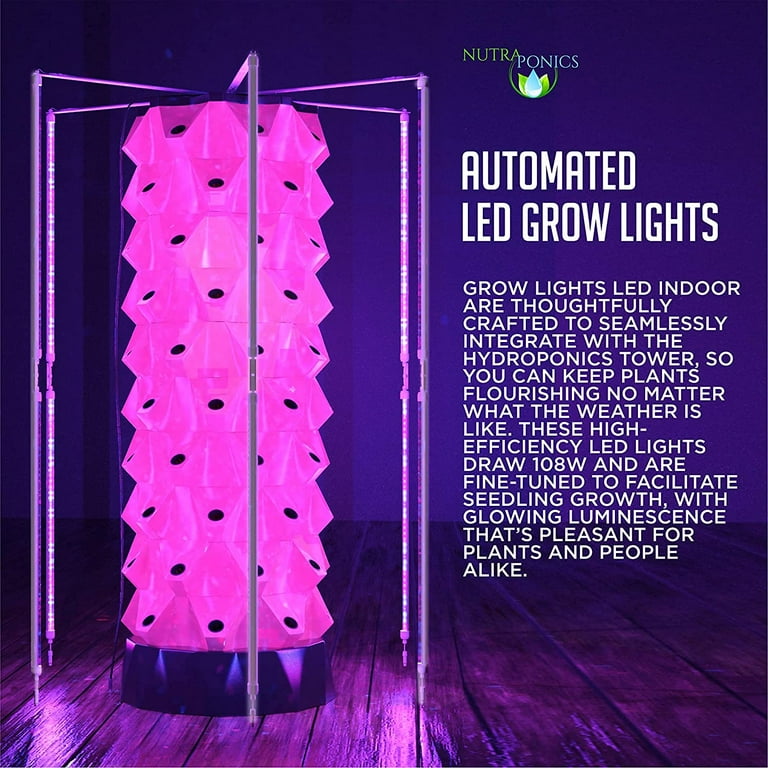The image is a square advertisement for Nutroponics automated LED grow lights, featuring a hydroponics tower. The background is predominantly dark blue, transitioning into a wooden floor at the bottom. The bottom left-hand portion is bathed in bright pink light, while the bottom right-hand area is engulfed in darker purples. Dominating the left side of the image, the brightly glowing pink tower stands on a black circular base. The tower, which appears textured and features interconnected metal beams, emanates a vivid pink and purple luminescence from multiple LED lights. At the top of the image, the word "Nutroponics" appears along with a graphic of a lily. The accompanying text highlights the high efficiency of these 108-watt LED grow lights, which are designed to seamlessly integrate with the hydroponics tower to ensure plants thrive regardless of weather conditions. The luminescence is noted to be pleasant for both plants and people.